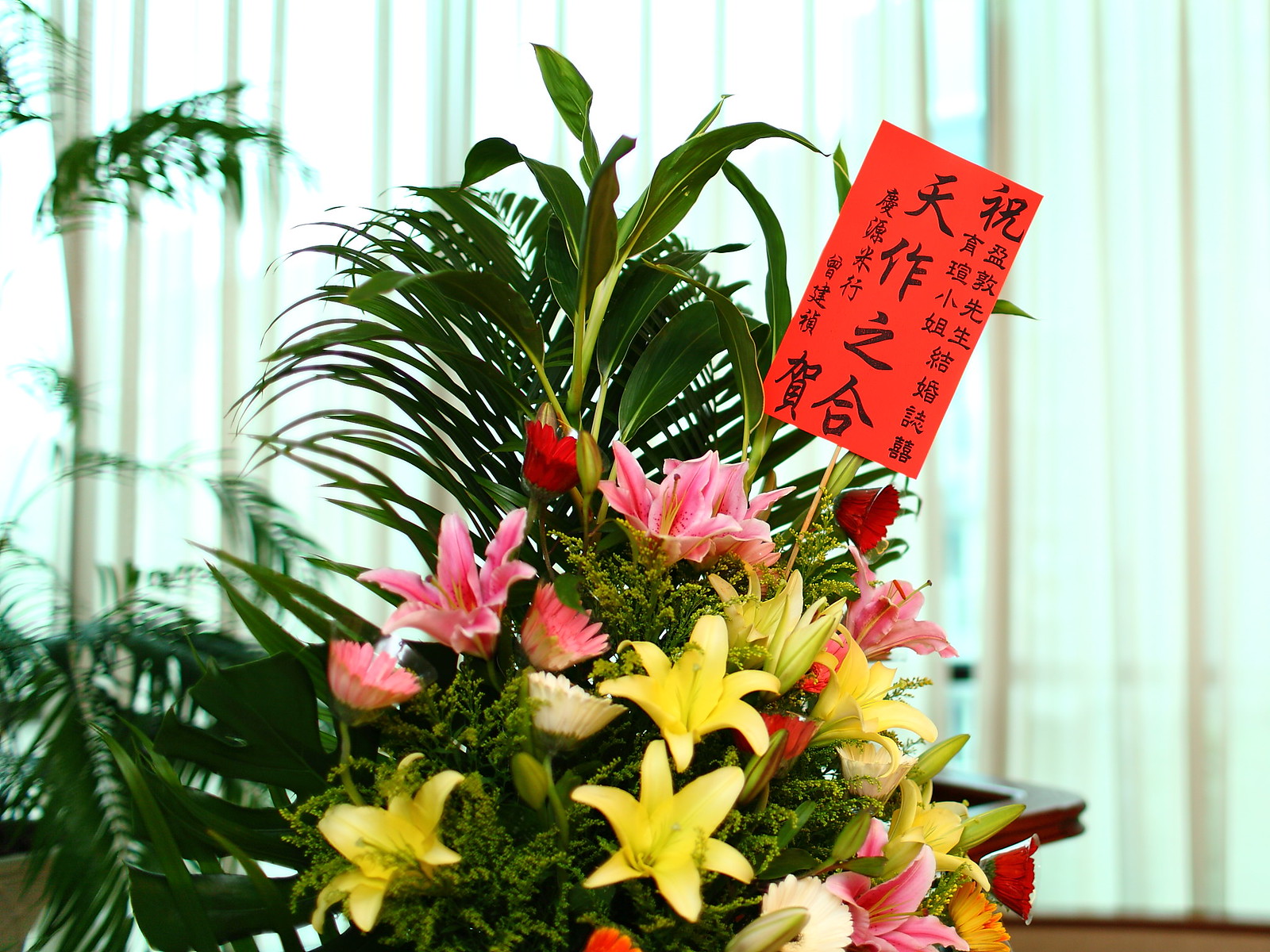This close-up image captures a vibrant flower bouquet against the backdrop of gauzy white curtains with sunlight streaming through. Prominent in this arrangement are the pink and yellow lilies, their long, pointed petals elegantly bending at the tips. Interspersed among these are red, orange, pink, and white daisies, and several striking red and orange gerbera daisies. The bouquet is enriched with abundant green foliage and delicate green buds, creating a lush, textured appearance. A small vertical card on a wooden skewer is embedded in the bouquet, featuring Japanese characters on a red-orange background. The floral arrangement is complemented by leafy ferns and other greenery, which add to its visual richness. In the background, partially obscured by the bouquet, is the corner of a wooden table.